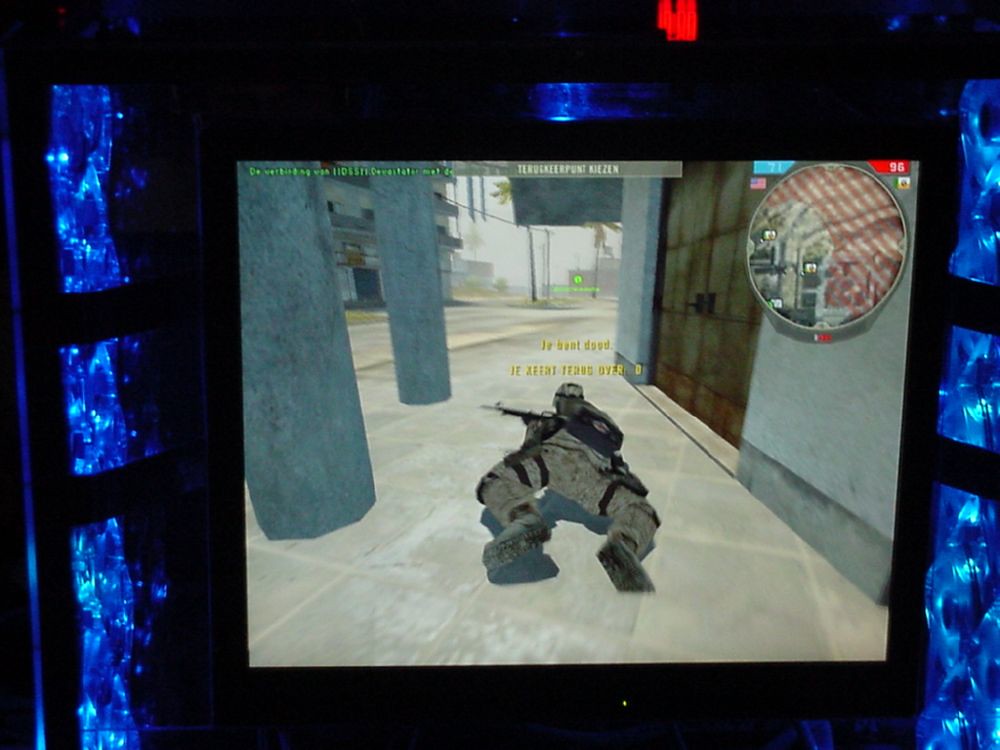In the video game image, there are distinct visual elements in various parts of the screen. On the very left and very right sides, there are structures resembling blue crystals or possibly see-through glass. At the very top, a red LED indicator is present, although its exact purpose is unclear. The central part of the image showcases an in-game character in a prone position, clad in a military uniform complete with leg straps, a helmet, and holding a rifle. The character also has a bag, and yellow text is displayed above them.

In the top right corner, there is a double door, while a scoreboard with some light blue labeling and red labeling is also visible, showing score numbers. Additionally, a mini-map is displayed, featuring terrain details. The top right diagonal section of the mini-map is marked with red dashes, possibly indicating an off-limit zone. The setting appears to include stone pillars, a stone floor, a visible street in the distance, and possibly some palm trees.